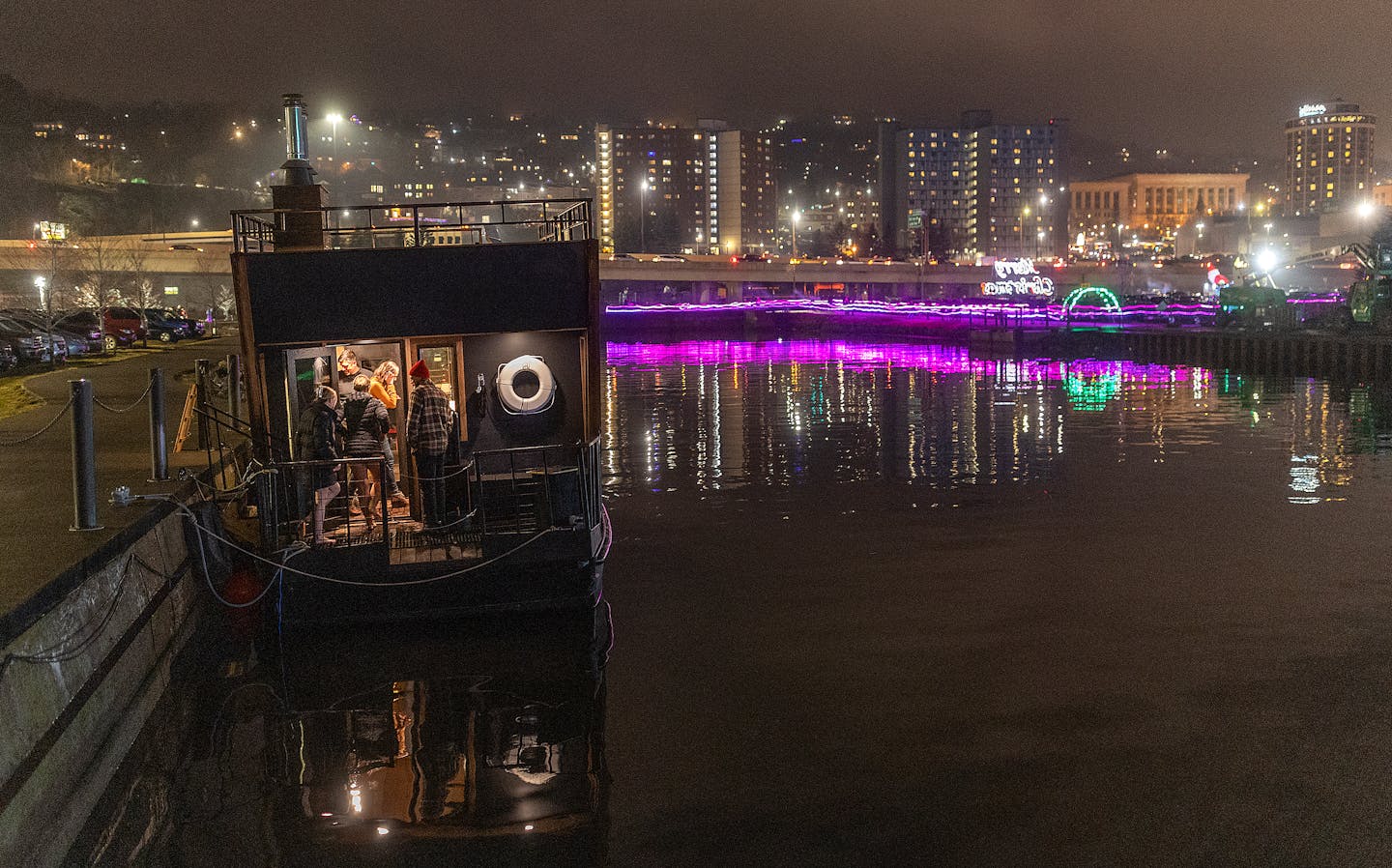The image captures a bustling nighttime cityscape featuring a skyline of tall, illuminated buildings, likely serving as either apartments or office spaces. These buildings, predominantly in shades of brown and black with some lighter structures intermixed, reflect their lights in a still body of water that occupies the foreground. The water is accentuated by neon purple and green lights that trace the perimeter of the city streets and an archway, producing a beautiful, colorful reflection. On the left side, a black houseboat is anchored against a dock framed by metal poles and chains. The houseboat shows signs of life, with several people visible both on the deck and inside. Notable figures include a woman with blonde hair in an orange shirt, a man in a red hat with a plaid shirt, a woman in a black coat, and another man in a striped jacket. In the vicinity, there's a parking lot filled with cars. The overall scene is lively yet serene, with the bustling city background contrasted by the calm, dark waters of the harbor.